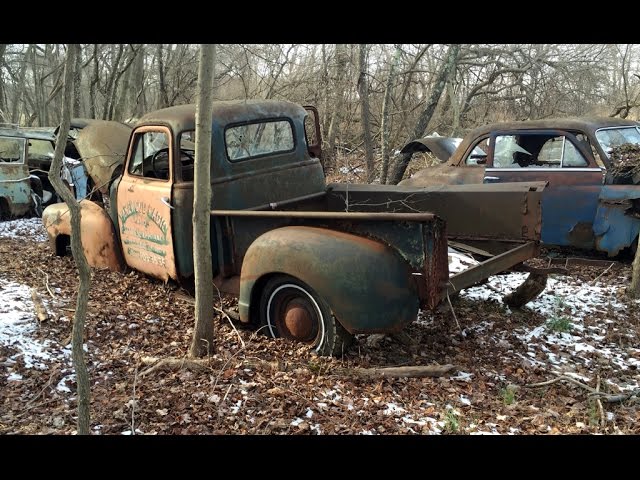Abandoned and weather-worn, this desolate scene captures an array of vintage vehicles nestled among the young trees of a wooded area, thick with fallen leaves and light patches of snow. Dominating the image is a rusted-out, 1950s-style pickup truck with a bulbous, endearing shape that hints at its once vibrant history. Its faded, rusty exterior, possibly once an orange-red shade, shows extensive wear; the hood is propped open, the bed has disintegrated, and the front tire is missing while the rear tire is half-buried in the dirt. The driver’s door, a faded cream color with an illegible graphic, adds a touch of past personalization. Adjacent to this central relic, another dilapidated vehicle that might have been blue stands with its hood crumpled and windows shattered. To the left, yet another rusted car peeks into the frame. Dead branches cover the ground, and all around, barren trees stretch toward a cloudy, overcast sky, enhancing the scene's melancholic beauty. The photograph, in a landscape orientation with black horizontal bars framing the top and bottom, epitomizes a representational realism style, precisely documenting this evocative moment of abandonment and decay.